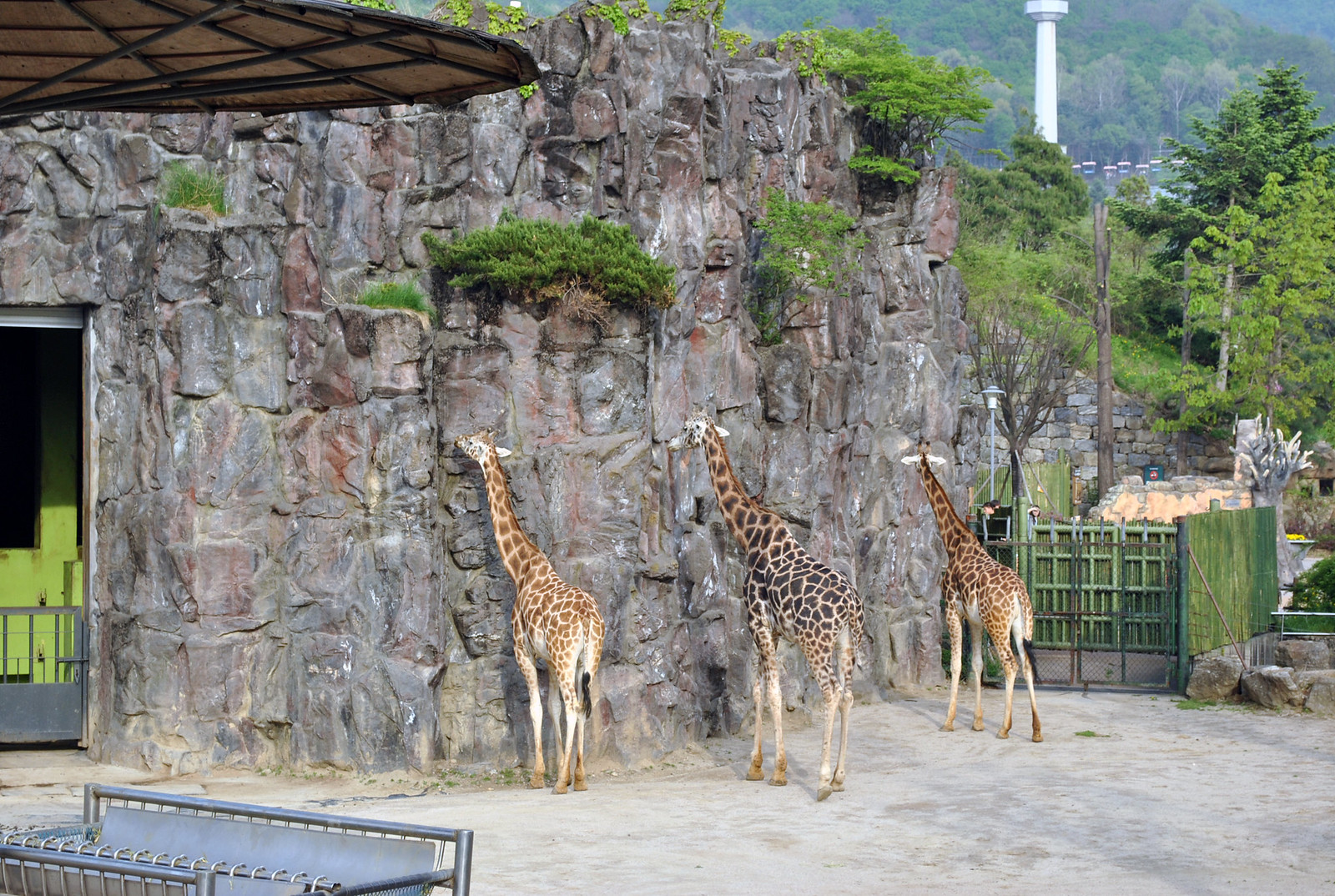In the zoo enclosure, the focal point is three giraffes facing and reaching up towards a large, man-made rock wall. The giraffes, with their distinct spotted coats—one noticeably darker than the others—appear to be foraging for food that may be tucked in the crevices of the rock surface. The artificial wall, resembling a mini cliff, is punctuated by an opening, perhaps for zookeepers' access, and flanked by a green fence or gate. In the background, lush green trees and mountainous regions visible beyond the zoo boundaries add a layer of natural scenery to the otherwise clearly constructed environment. A metal apparatus and some sort of green structure, possibly holding food, are also visible near the enclosure. The overall setting, though filled with greenery and rocky elements, unmistakably reflects a man-made habitat designed to house and care for these towering animals.